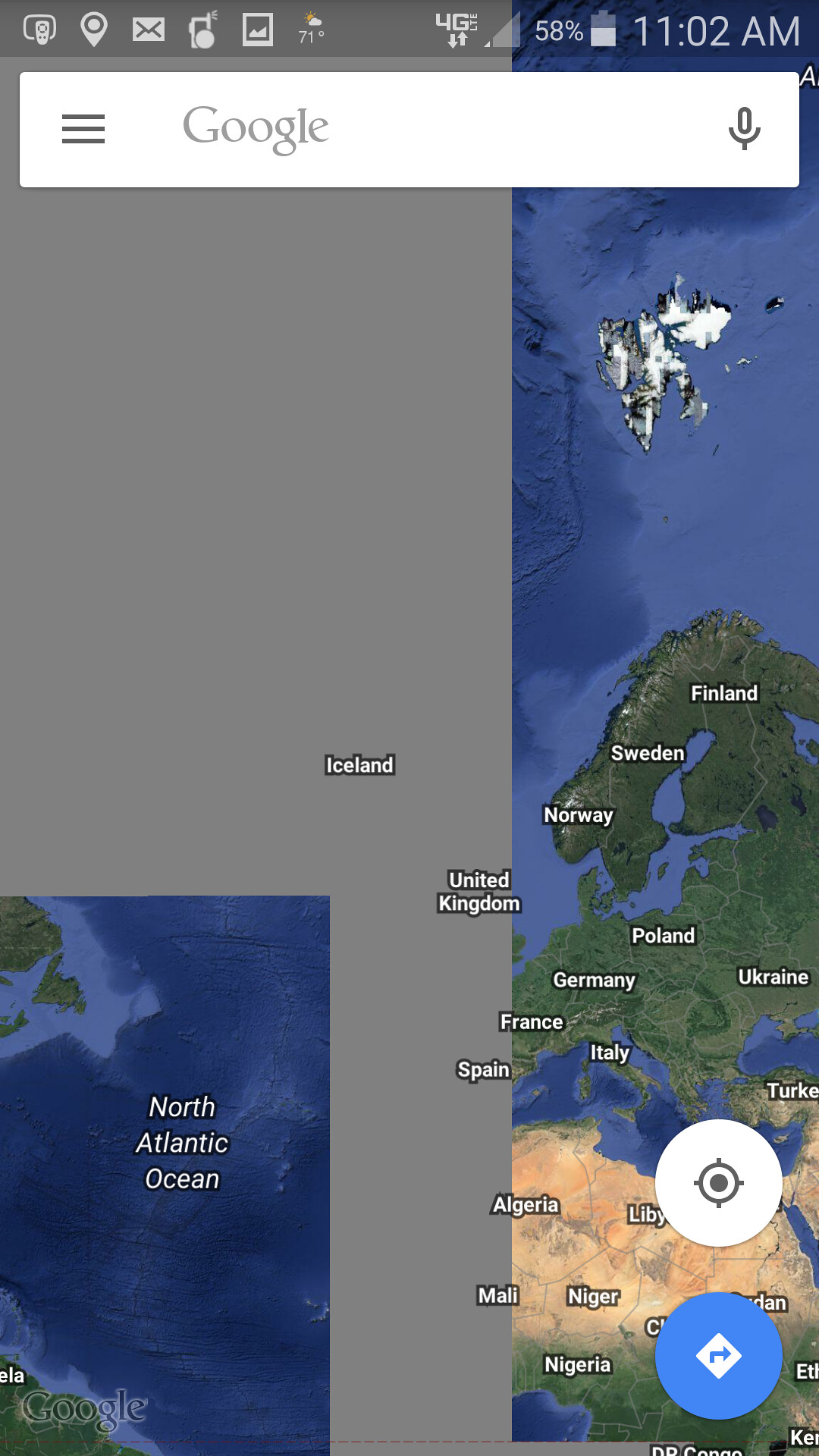This screenshot displays the Google Earth interface on a mobile phone, as seen through various UI elements at the top, including the time, battery icon, the 4G logo, and multiple app notification icons. At the very top, a Google search bar remains untyped. The central focus of the image is a map showcasing Europe and the northern part of Africa, with the Atlantic Ocean dominating the center. Significant portions of the map, especially areas west of France and parts of Africa, are obscured by gray squares. The map visually distinguishes regions with color coding: European countries in green, and the northern part of Africa in yellow to depict the desert. Faint borders mark country divisions, with countries like Finland, Sweden, Norway, Poland, Germany, Spain, Italy, Turkey, Ukraine in Europe, and Algeria, Mali, Niger, Nigeria in Africa being identifiable. The map also features labels for North Atlantic Ocean in white text. In the lower left corner, there's a Google watermark, while the lower right corner includes a blue circle with a turn arrow and a white circle with a gray crosshair icon above it.